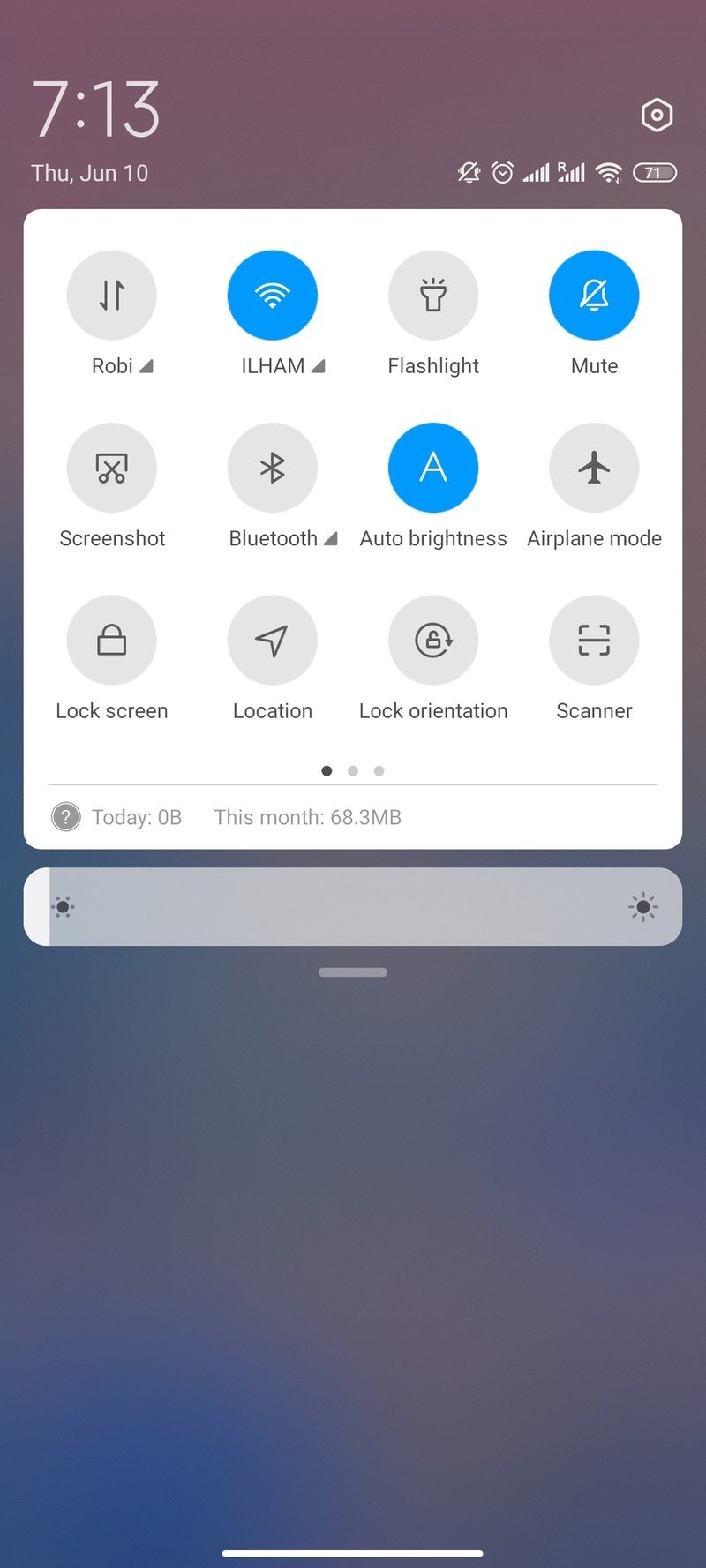In this detailed screenshot, we observe a user’s phone notification panel, meticulously timestamped at 7:13 on Thursday, June 10th. The panel is captured from the upper left corner of the display. On the top right, a settings gear icon is prominently visible, with the battery level indicating a remaining charge of 71%.

Dominating the scene is a compact, white control square, featuring multiple operational buttons labeled: Robi, ILHAM, Flashlight, Mute, Screenshot, Bluetooth, Auto Brightness, Airplane Mode, Lock Screen, Location, Lock Orientation, and Scanner. Out of these controls, only ILHAM, Auto Brightness, and Mute are enabled, distinctly highlighted by blue circles, contrasting against the inactive gray buttons.

Beneath this control square is a horizontal slider bar, ostensibly for adjusting the screen brightness. The slider is minimally adjusted, just slightly filled in on the extreme left, indicating low brightness.

The background of the image is mostly blurred, suggesting a glimpse of the user’s home screen, yet leaving it indistinct and unfocused.